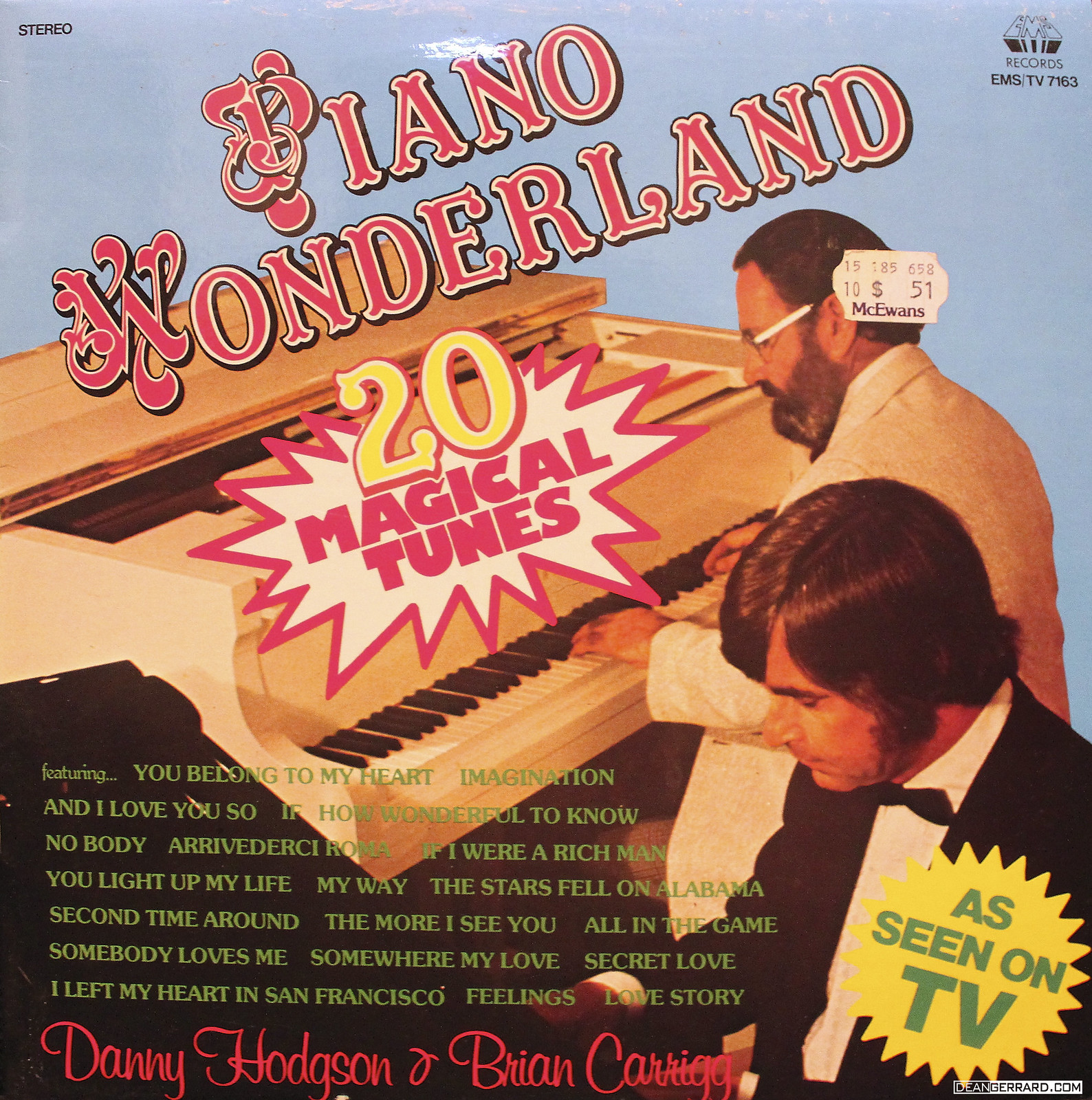The image showcases a vintage record album cover, distinguished by its square format and aged appearance. Dominating the top section, angled skyward, is the title "Piano Wonderland" inscribed in a red stylized font with decorative capital letters, bordered by yellow and black. The background is a clear, inviting sky blue. Centered below this title is a tan grand piano keyboard, which a burly, bearded pianist with short dark hair, glasses, and dressed in a light beige blazer is playing. A striking white and red starburst above the keyboard announces "20 Magical Tunes," with the number "20" highlighted in gold.

In the foreground on the bottom right, another musician stands in a black tuxedo, complete with a white shirt and bow tie, looking downward. He sports long brown hair and prominent sideburns. A yellow starburst to his side exclaims "As Seen on TV." The bottom left section features six lines of titles for the musical numbers in light green all-caps script, set against a darker background. Prominently displayed near the bottom are the artist names "Danny Hodgson and Brian Kerrig" in bold red letters. Additionally, the top right corner bears a price sticker, identified as "McEwen's 51 cents," further emphasizing the vintage nature of this album cover.